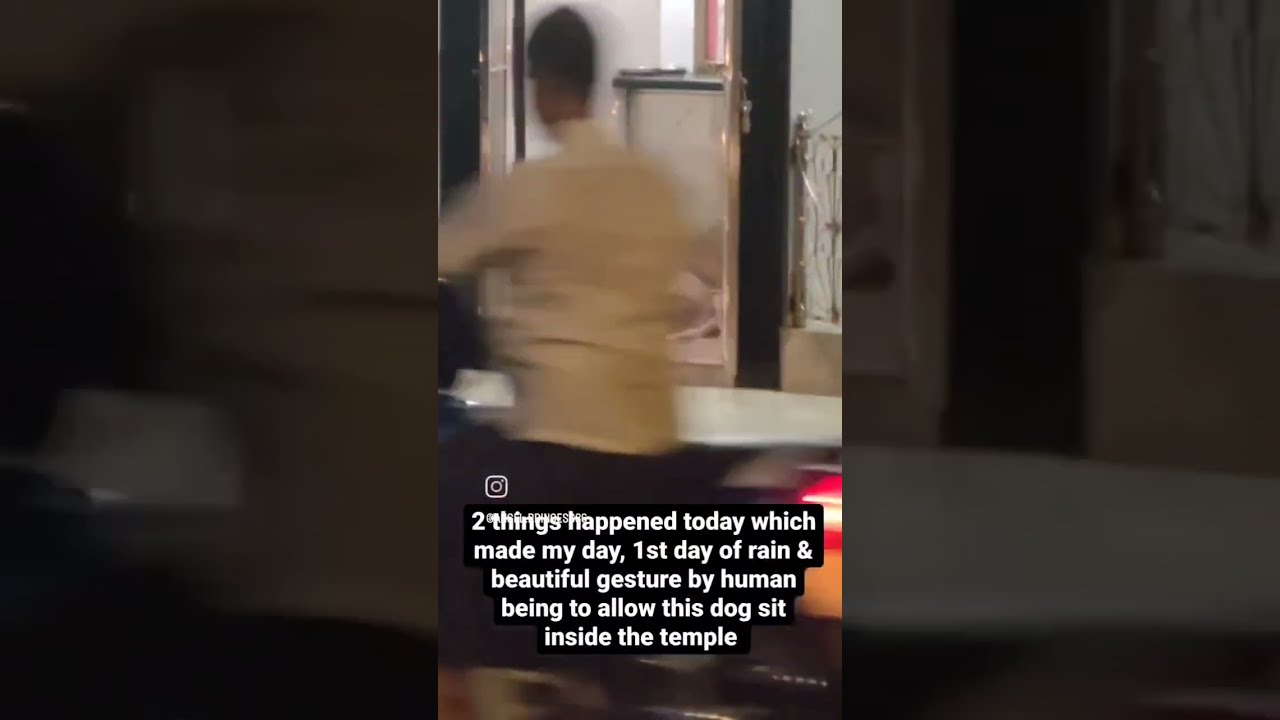The image shows a blurry photograph of a man in motion, positioned directly in the center, wearing a white dress shirt and dark pants. His upper body and face are obscured, suggesting movement. The scene includes multiple objects at the top of the screen, potentially a mirror or some other reflective surface, and he seems to be in an environment that could either be a bathroom or a temple, although no dog is visible as mentioned in the text. There is a suggestion of a metal gate or doorway with a railing to the right. The photo includes text at the bottom in white lettering on a black background, stating, "Two things happened today which made my day. First day of rain and beautiful gesture by human being to allow this dog sit inside the temple." The colors present are a mix of black, white, gray, red, and orange. The overall appearance suggests the image may be a screenshot from a social media app like Instagram or TikTok, evidenced by the layout and possible logo. The image structure consists of three panels, with the outer panels magnifying portions of the central blurred image.